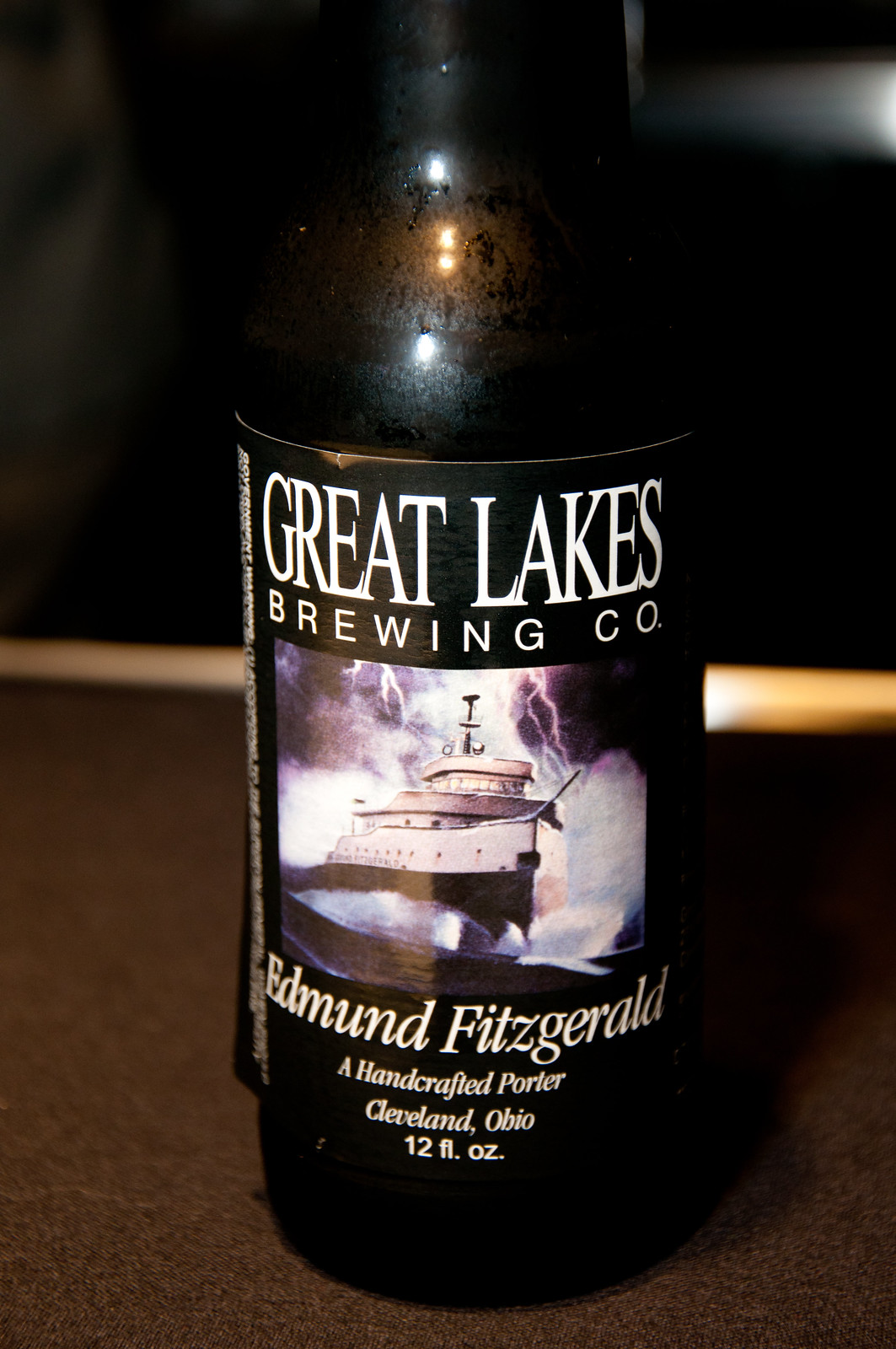The image depicts a dark glass bottle of Great Lakes Brewing Company beer, specifically their "Edmund Fitzgerald" handcrafted porter. The label prominently features the brewery's name in white text, along with an intricate illustration of a ship navigating through a storm, complete with lightning, turbulent ocean waves, and roiling clouds. Beneath the ship, the label denotes the beer's name, "Edmund Fitzgerald," followed by its description as a handcrafted porter and its origin in Cleveland, Ohio, along with the volume of 12 fluid ounces. The bottle appears chilled, evidenced by the condensation and water droplets on its surface. The setting of the image is quite dim, with the bottle resting on a brown, cloth-like surface. In the background, there is a light brown pool stick laying flat on the table, and a white blur is visible in the top right corner, adding an additional element to the scene.